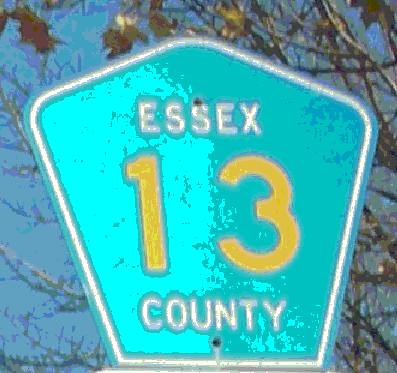This image is a close-up of a distorted, pentagonal road sign with rounded edges and a slightly unusual shape that includes a triangle-like protrusion at the top. The sign features a color scheme dominated by bright teal and turquoise for its background, with white capital letters reading "Essex County" and large yellow numerals "13" in the center, clearly indicating County Route 13. It also has a white border running around its perimeter. The sign is mounted on a pole that isn't visible in the photograph; however, two dark brown or blackish screws securing it to the pole can be seen. The photograph appears to have been taken from a low angle, looking up at the sign against a blue sky. The background features bare tree limbs with a few brown and dying leaves, along with some green leaves, suggesting the sign is located near trees. The entire image has a grainy, posterized look, as if filtered. This scene is bathed in bright light, hinting at a summer afternoon setting.